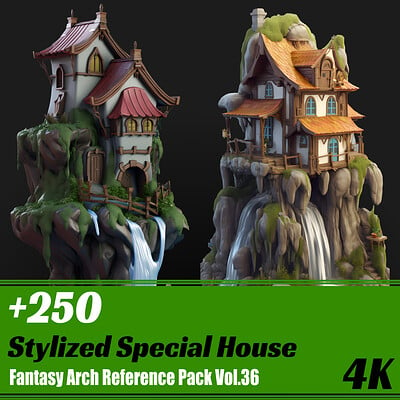The advertisement image on a black background prominently features white and black text, reading "Stylized Special House, Fantasy Arch Reference Pack, Volume 36," with "4K" in the bottom right corner. The design showcases two distinct, animated or cartoon-like houses set against green, brown, and mossy hillsides. 

The house on the left appears to be a whimsical, ceramic fantasy structure with a multi-tiered design. It features an arched entryway, multiple doors, and various forms of awnings; one is red and overlooks the windows, and the other peaks into a brown roof with a gray tower section, complete with another peaked brown roof. A charming waterfall cascades down beside this tree-like and brown house, which has small yellow windows and a vividly white exterior crowned by a red roof.

The house on the right possesses a contemporary aesthetic with a flat front, red awning, blue door, and yellow sides. It sits proudly atop another mossy hill, having a slightly different, yet similarly colorful design. This structure maintains symmetry with a porch or entryway on its left side and features a slanted roof, V-shaped window, and a gray chimney at the top left. Both houses exude a fantasy ambiance enhanced by flowing waterfalls.

The green overlay bar at the bottom of the image emphasizes the collection's unique and stylized architectural references, suggesting a vast pack of 250 high-definition animated house designs, ideal for fantasy settings.